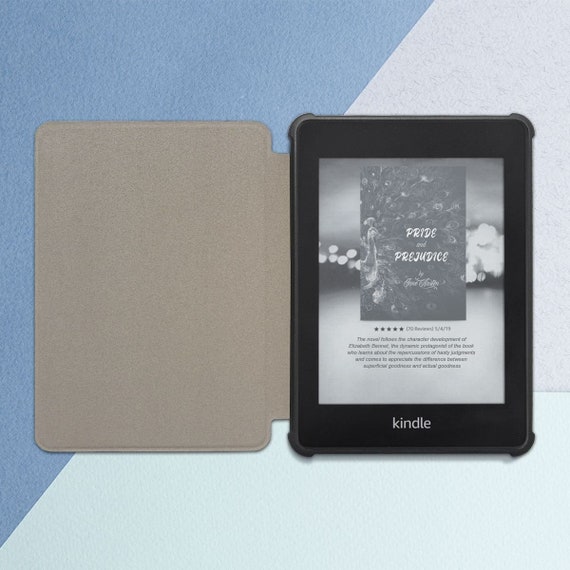The image depicts an Amazon Kindle e-reader situated against a segmented, colorful background. The background features a blend of solid colors starting from a darker denim blue on the left diagonally transitioning to sky blue at the top right and a greenish robin's egg blue towards the bottom, accented by blurs of light adding depth. The Kindle is open with its grey, leathery protective cover flipped to the left, exposing the screen and black plastic frame of the device. On the bottom of the Kindle's black frame, the word "Kindle" is prominently displayed in white. The screen, in black and white, shows the cover of "Pride and Prejudice," recognizable by its detailed design, which some describe as looking like a peacock. Below the book cover, there are five black stars, hinting at a high rating, though the accompanying text is too small to read.